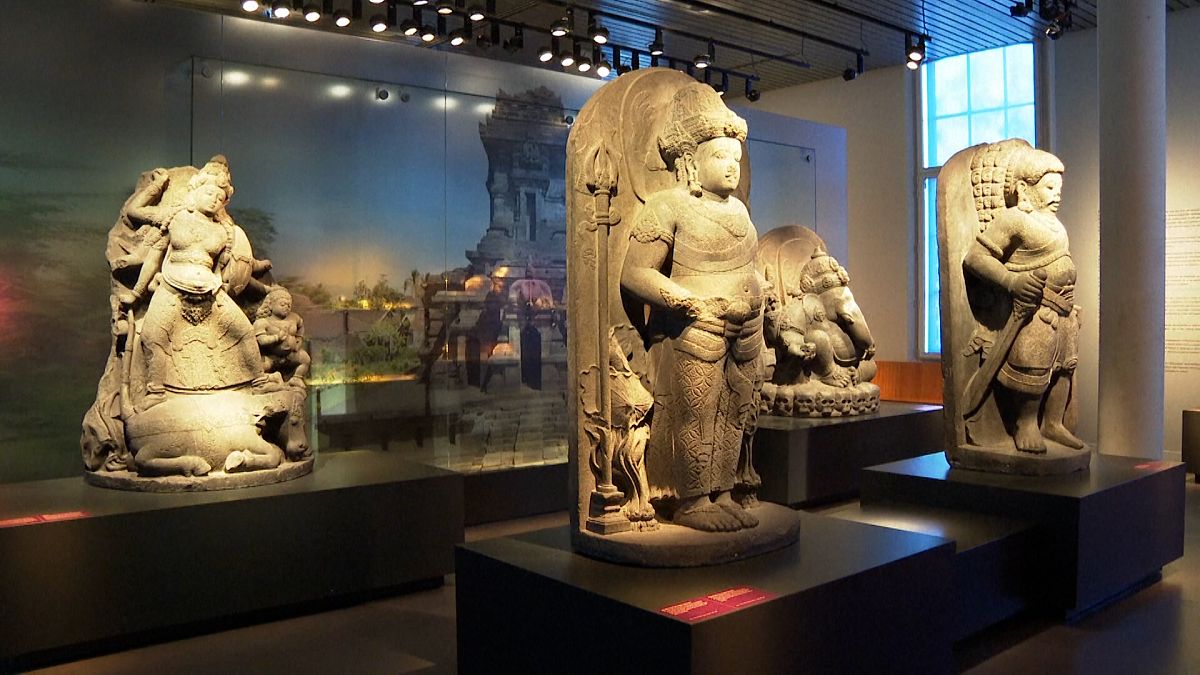In this photograph, set within a museum or display area, four intricately carved stone statues are prominently featured, each exuding an air of historical and cultural significance. These statues appear to be from an ancient Oriental or Asian era, possibly of Mongolian influence, reflected in their distinct attire and headgear. 

The first statue, positioned at the front, appears to be a warrior standing upright, with hands resting near the hips, adorned with a high, stylish headdress. To the left of this figure stands or sits another statue, which seems to depict a woman, notable for its feminine features and stylized representation. Further left, there is a unique statue, distinct for including both an adult and a child, adding a familial dimension to the display.

The most rearward statue in the right corner is of a warrior, distinguishable by a large and thick sword held in his right hand, pointed downwards. This figure wears no headdress but instead has a mask obscuring its features, making it appear enigmatic. Both this warrior and the one in front are depicted with bare feet, a detail that adds to their intriguing and somewhat stylized portrayal. 

Behind these statues, the backdrop consists of ambient lighting that highlights each figure and a mural depicting a historical castle, enhancing the overall atmosphere of antiquity and martial heritage. The display evokes a sense of reverence for the past, capturing the essence of ancient warriors poised in enduring silence.